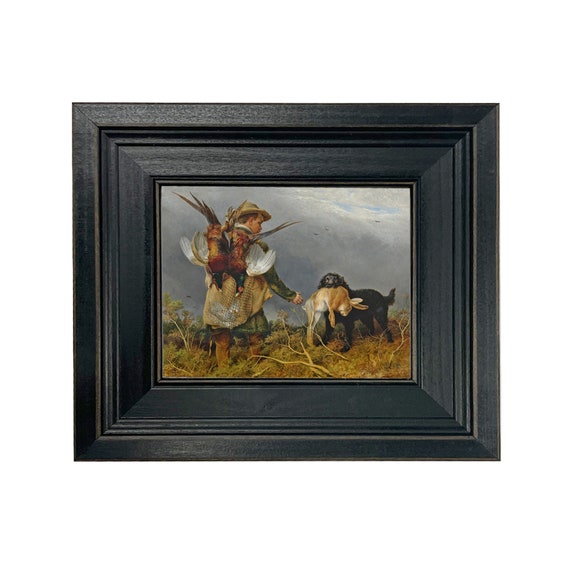This detailed painting, surrounded by a thick, black wooden frame with a large flat edge and receding inner area, showcases a hunter and his black Labrador retriever in an outdoor, marshy field with tall grass. The hunter, a Caucasian male, is dressed in an olive-green jacket, brown boots, and a khaki-colored hunting hat with a brim. He stands with his back to the viewer, extending his right hand towards the dog. Over his shoulder, he carries two pheasants, characterized by their green necks, dark heads, and speckled or striped feathers. The dog holds a light brown rabbit in its mouth, facing the viewer. The painting's background features a darker, cloudy, and windy sky, adding to the overall atmospheric depth of the scene. The artwork utilizes a color palette that includes shades of gray, black, tan, beige, white, green, dark brown, and light blue.